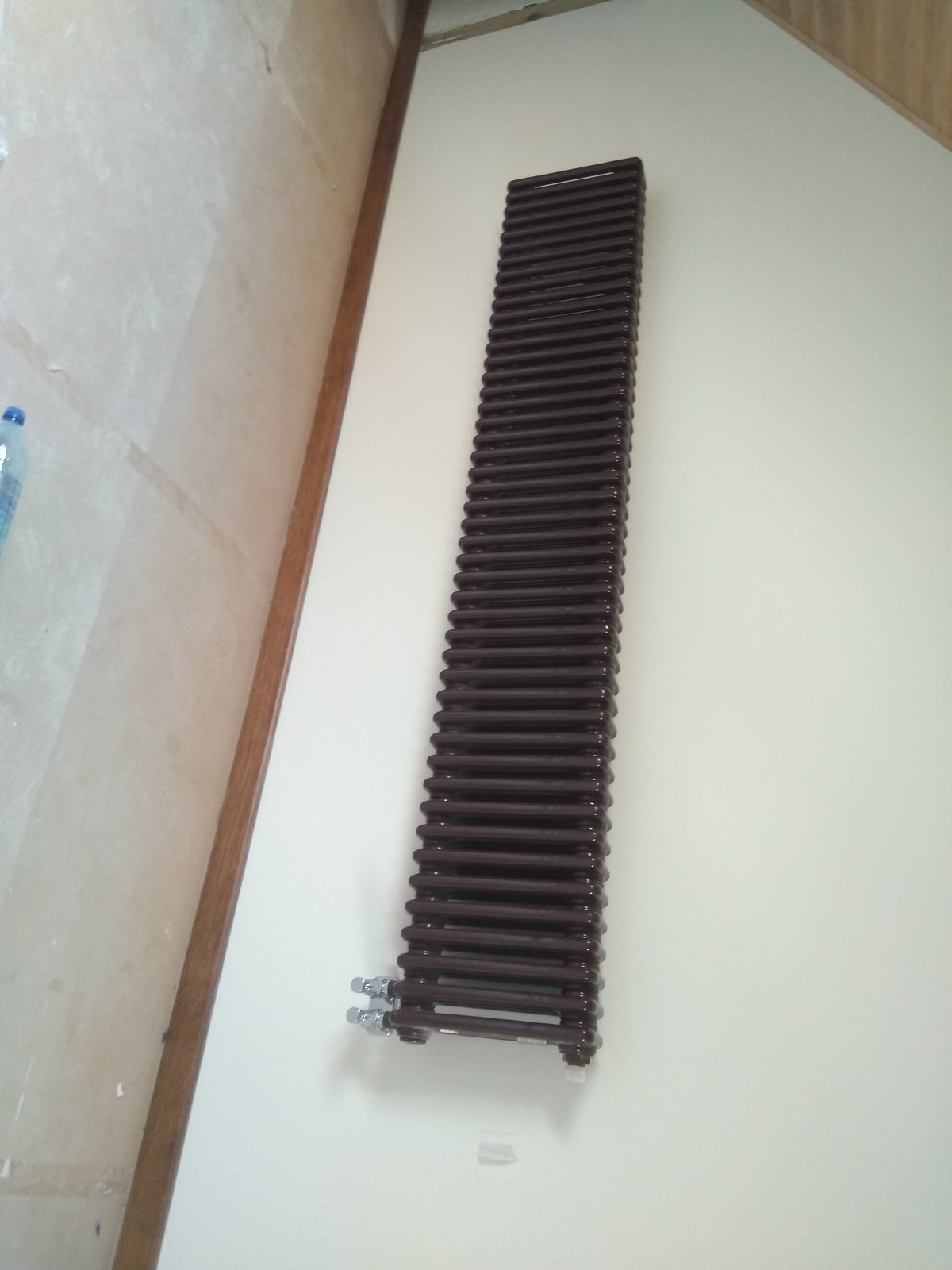The image appears to show a mixed area with distinct sections and diverse materials. On the left-hand side, we see what seems to be a dark white tile transitioning into a tan color, which then meets a segment of wood. Just beyond this wooden section is a white area, no longer tiled, that appears to border a darker baseboard running from the top towards the bottom left of the image, creating a sense of segmentation. The upper right-hand corner features a triangle of light brown wood with outlined edging.

In the middle, there's a curious black object that resembles a radiator with vertical elements and silver metal tips or clear plastic tips on the left-hand side at the bottom. Some describe it as possibly composed of black lines or pipes. A blue water bottle is partially visible on the upper left-hand side of the image, while the overall flooring looks like a laminate material in various shades of gray with brown lines separating the segments, giving the image a structured, yet complex composition.